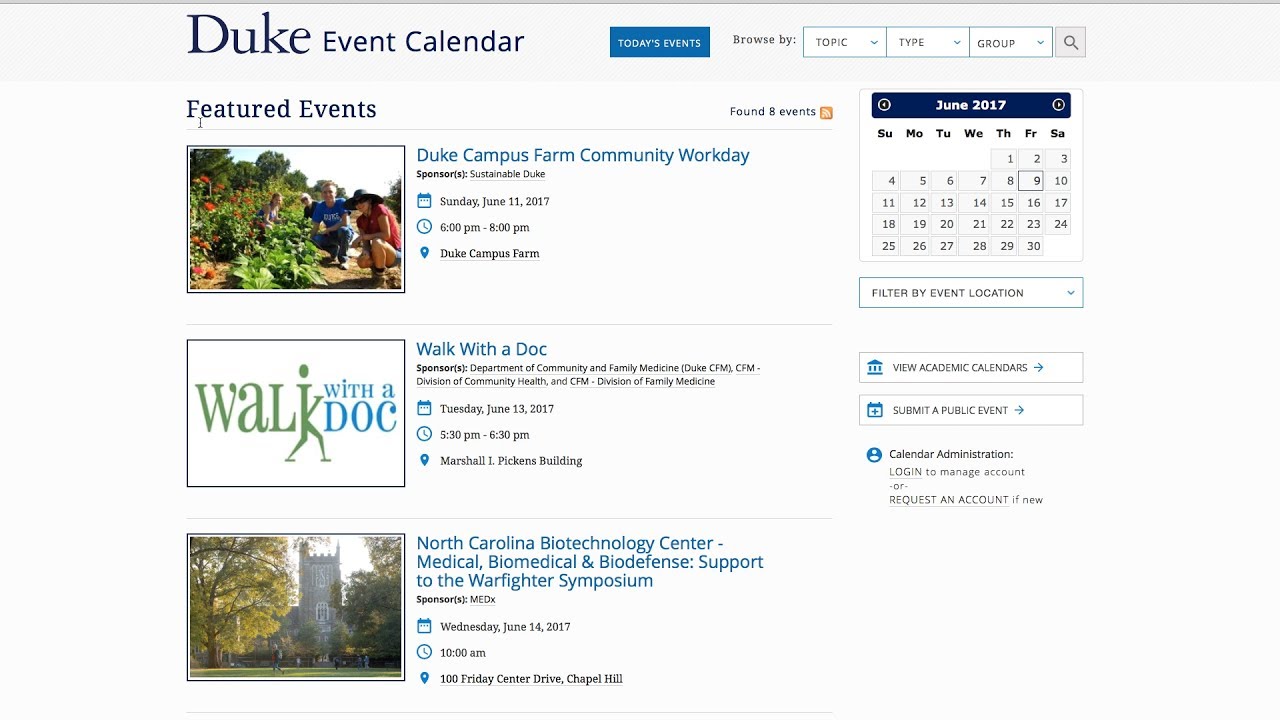The image is a detailed screenshot of a Duke Event Calendar webpage. At the top of the page, a gray bar spans horizontally with the text "Duke Event Calendar" prominently displayed in blue. Below this, there's a blue button labeled "Today's Events." Adjacent to it is a section labeled "Browse By" with three drop-down buttons for navigating events by "Topic," "Type," and "Group." A search icon, depicted as a magnifying glass, is also present for keyword searches.

Further down, the section titled "Featured Events" is highlighted in blue font. The interface indicates that eight events have been found. To the right, there is a calendar displaying the month of June 2017, with June 9th highlighted.

The list of events begins with a blue hyperlink reading "Duke Campus Farm Community Work Day," accompanied by an image showing four individuals standing in a garden area. This event is scheduled for Sunday, June 11th, 2017, from 6 p.m. to 8 p.m. at Duke Campus Farm, and it is a sponsored event.

Another event listed is "A Walk with a Doc," scheduled for June 13th, 2017. The text and layout offer a clear and organized view of upcoming activities on the Duke campus, providing users with multiple ways to explore and engage with event information.